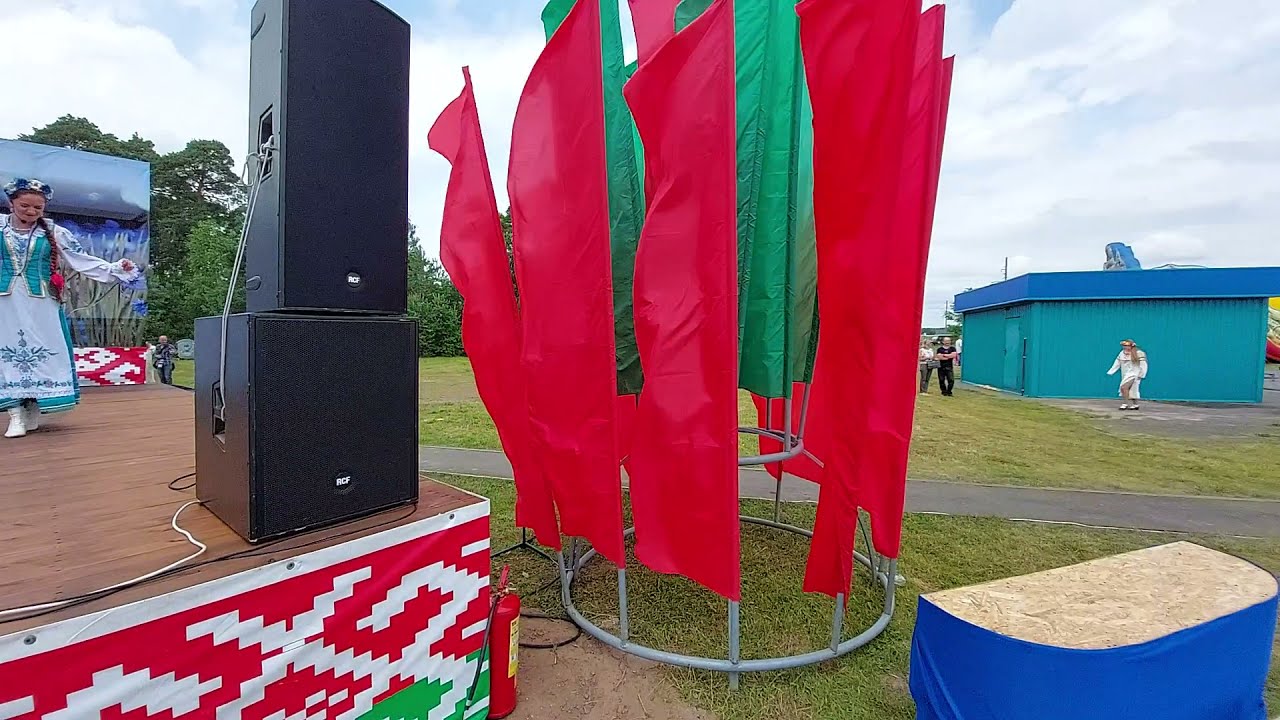The image captures an outdoor scene of a Scandinavian celebration in a city park on a cloudy day. In the foreground, a wooden stage is situated on the left-hand side, adorned with a decorative cloth that features red and green stripes with intricate white patterns. Dominating the stage are two large speakers, a rectangular one perched atop a square one. Behind the speakers stands a young girl with braided hair, dressed in a traditional Scandinavian outfit that includes a white dress with a green vest and patterned details. Adjacent to the stage is a metal structure displaying long rectangular flags with green centers and red edges. Beyond the stage, an outdoor building appears, its base painted teal green and its upper section a shade of blue. Surrounding the scene is a lush, well-trimmed grassy expanse intersected by a thin paved walkway, with deciduous trees visible in the far background. Additional details include people walking around the park and the presence of a blue covering on a flat-topped structure to the right of the flags.